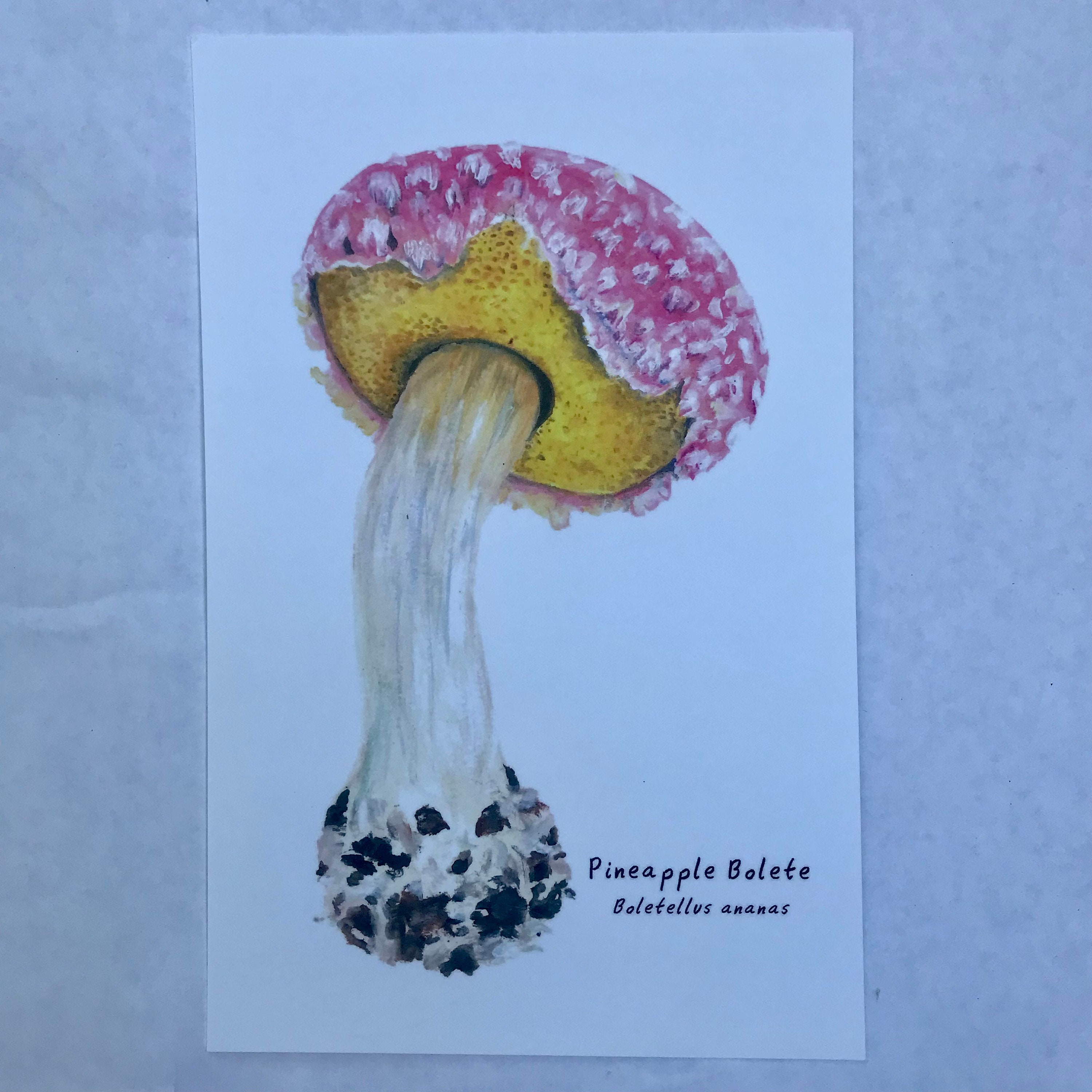The image depicts a hand-drawn illustration of a mushroom on a white piece of paper, which is either lying on a white table or possibly affixed to a wall with a grey or bluish tint. The mushroom, identified as "Pineapple Bolete" with the scientific name "Boletulus ananas" written in black text at the bottom right of the paper, features a distinctive elongated stem and a large cap. The stem appears to be white and somewhat transparent, with black and grey areas near the base, suggesting it might have been freshly pulled from the soil. The cap of the mushroom boasts a spongy yellow underside rather than gills, and the top surface is marked by a vibrant mix of pink and yellow, adorned with white dots, giving it a scaly or dotted pattern. The detailed illustration highlights the unique characteristics of the mushroom, showcasing artistic strokes that imply it was painted by hand.